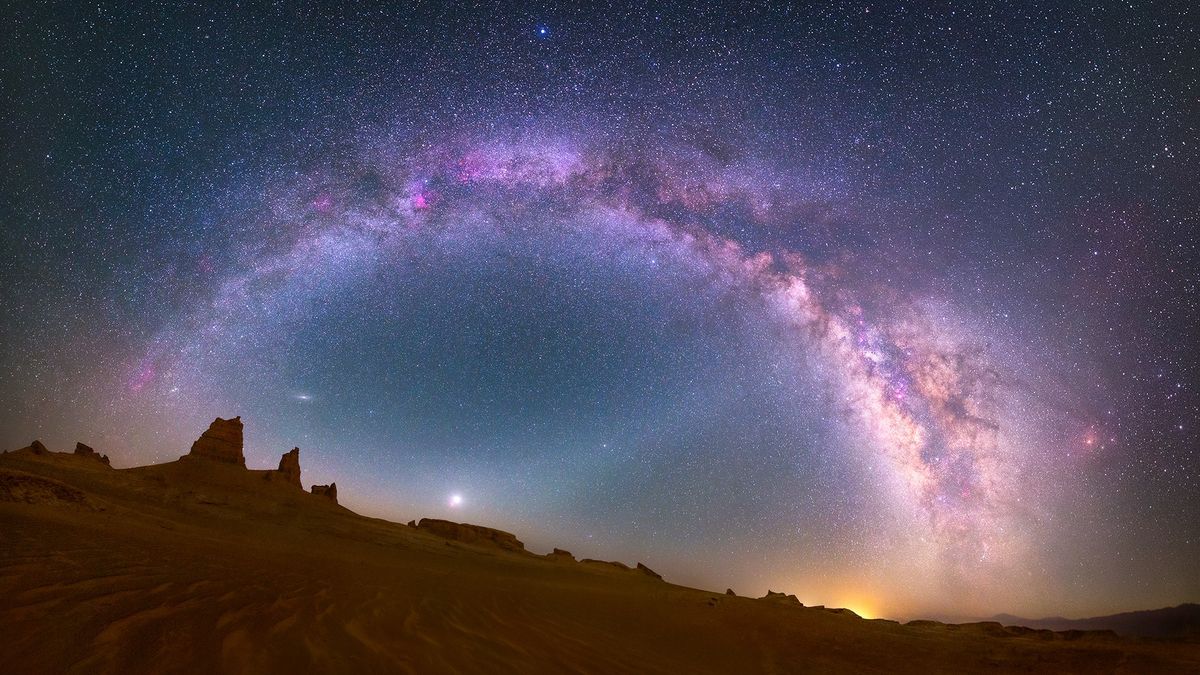The image captures a vivid night sky, with a breathtaking display reminiscent of the Aurora Borealis, blending hues of purple, pink, blue, and a touch of yellow near the horizon. The darkness of the vast expanse is dotted with countless stars, some appearing closer and brighter than others. A curious, bright spot, possibly the moon, adds to the serene ambiance. Ethereal clouds or vapor arcs across the sky, creating a peaceful, restful scene. The foreground hints at a desert landscape featuring subtle reddish-brown sand and rock formations. This picturesque view, possibly depicting an otherworldly landscape, showcases the pure beauty of the night sky in the desert.